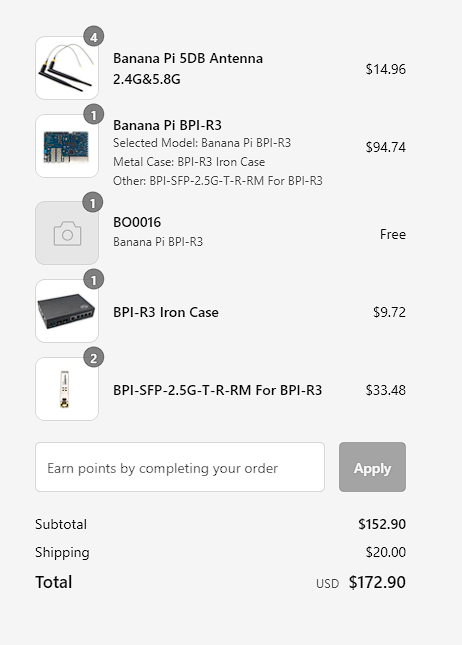This vertical image features a predominantly medium gray, flat background with no visible texture, creating a one-dimensional appearance. At the top of the image, there is a dark gray circle with the number 4 inside, rendered in white. Beneath this, there is text that reads "Banana Pi 5dB Antenna 2.4G and 5.8G 1496."

As we move down the image, we encounter several rectangular sections:

1. The first section displays a gray circle with the number 1 inside. The text here reads "Banana Pi BPI-R3" in bold, followed by "Selected model: Banana Pi BPI-R3," "Metal case: BPI-R3 iron case," and additional alphanumeric codes. The price listed is $94.74.

2. The next section also includes a gray circle with the number 1. This one contains a picture of a camera and the code "BO0016 Banana Pi BPI-R3," labeled as free.

3. Another section shows a gray circle with the number 1, featuring the "BPI-R3 iron case," priced at $9.72.

4. Further down, a gray circle with the number 2 is shown, accompanied by another string of letters and numbers, listed at $33.48.

Toward the bottom, there's a white box containing the text: "Earn points by completing your order. You can press apply." Below this, the subtotal is shown as $152.90, shipping is $20, leading to a grand total of USD $172.90.